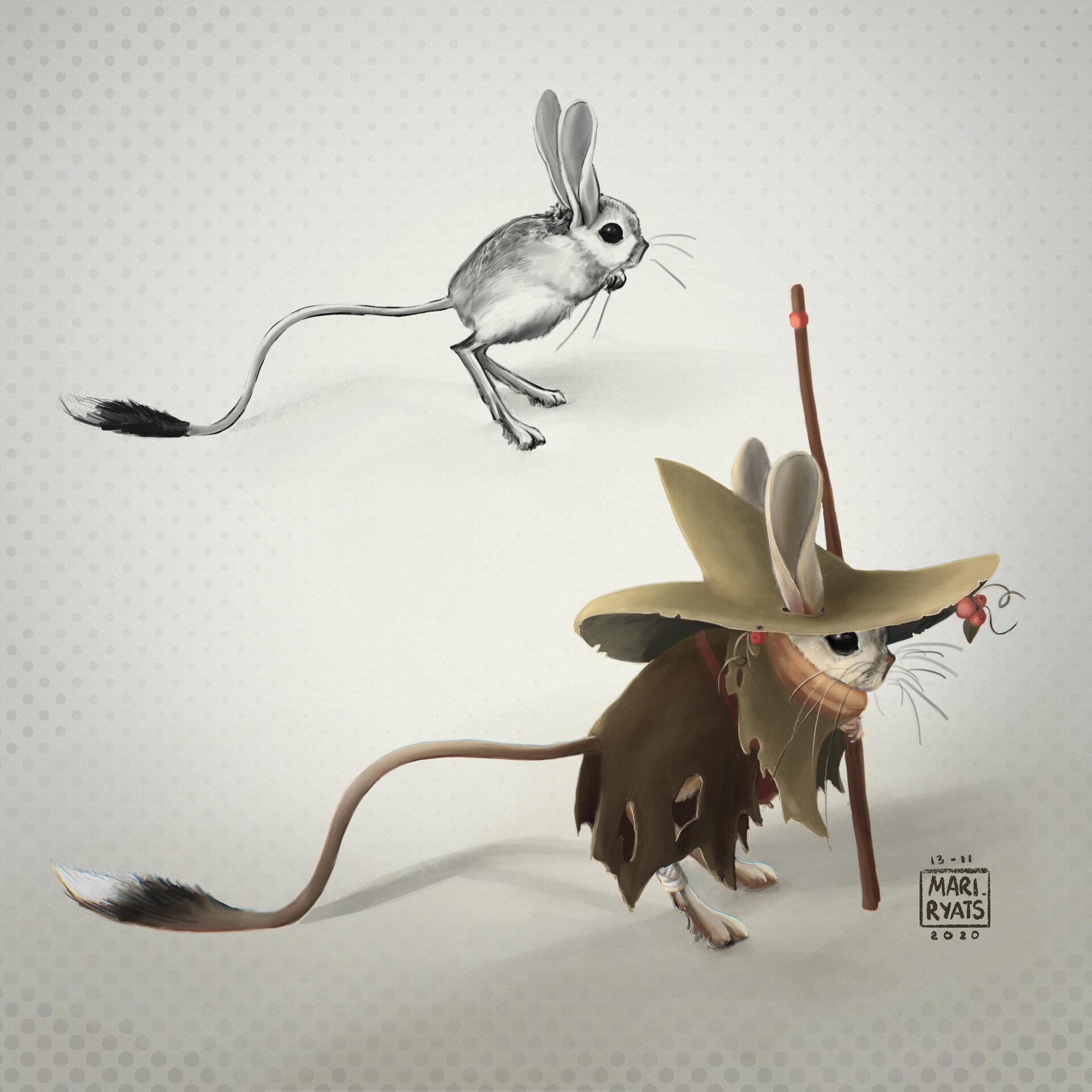The image features two representations of a fantastical rodent character with large ears, standing on its rear legs. In the background, a black-and-white, two-dimensional sketch of the character is visible. This version showcases the rodent with its characteristic long tail, which has a black tuft at the end and a white tip, large dark eyes, and long whiskers. The rodent in the foreground, however, is depicted in full color and more detail, giving it a three-dimensional effect. Dressed in a tattered, dark brown wizard-like robe and shawl, the character also wears a beige hat with holes for its ears and a matching scarf. A white bandage is wrapped around its leg. The rodent holds a wooden walking stick and stands upright, gazing to the right. Its attire, including the hat and scarf, are tattered, adding to its hobo-wizard aesthetic. At the bottom right of the image, the signature "MARIE WRIGHT, 13-11-2020" is inscribed.